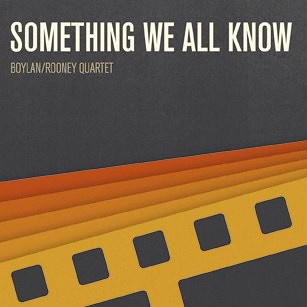The image is a perfect square with a predominantly black background. At the top, in bold, white, capital letters, it reads "Something We All Know." Below this title, in smaller capital letters, it says "Boylan/Rooney Quartet." The bottom half of the image features a series of horizontal stripes, transitioning from red at the top, to dark orange, lighter orange, and finally yellow. The lowest yellow stripe is thicker and contains five small black squares, arranged in a line that ascends slightly from left to right, stopping near the center of the image. The overall design suggests it could be an album cover, given its simplicity and the arrangement of text and colors.